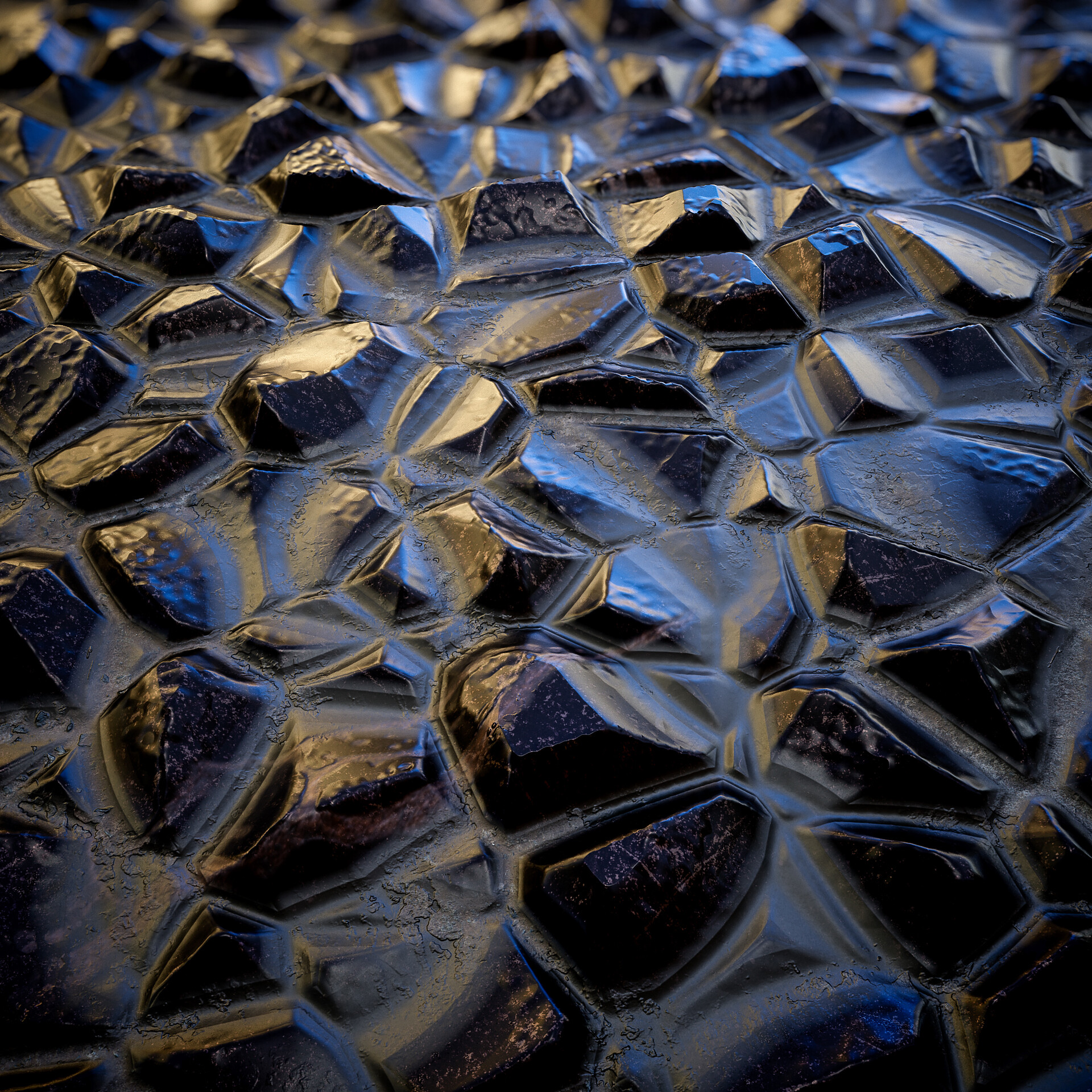The image showcases a close-up view of numerous jet black, semi-gloss polished stones, arranged in a pattern reminiscent of a soccer ball, creating a blanket-like structure. These stones appear to be onyx or a similar dark mineral, and their surfaces exhibit a series of bumps and raised areas. There is water partially submerging some of the stones, giving them a slick and slightly shiny appearance. A light source from the top left of the image creates sheens and shines across the stones, enhancing their glossy and polished look. The composition suggests a total of approximately 25 to 40 individual stones, each catching the light in a way that highlights their unique micro-textures and subtle variations in sheen.